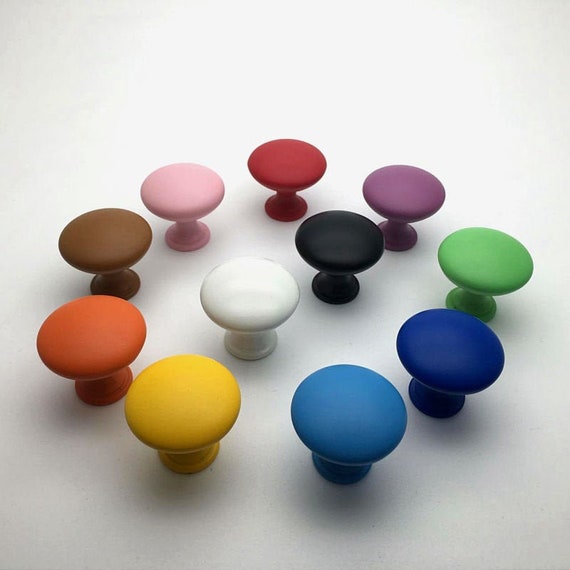This image features a variety of colorful objects arranged in a precise circular pattern against a predominantly white background that transitions to gray at the bottom. The objects, which could be interpreted as either doorknobs or stools, stand upright with their larger, smooth, and possibly handle-like parts pointing upward. Encircling the composition are doorknobs in striking hues: orange, yellow, light blue, dark blue, green, purple, red, pink, and brown. At the center of the circle, two contrasting doorknobs—one black and one white—stand out. The lack of surrounding objects makes it difficult to ascertain their true size, leaving some ambiguity as to whether they are doorknobs or perhaps small chairs, given their resemblance to mushrooms. Additionally, subtle shadows cast by the objects add a delicate depth to the otherwise minimalist and professional photographic setup.